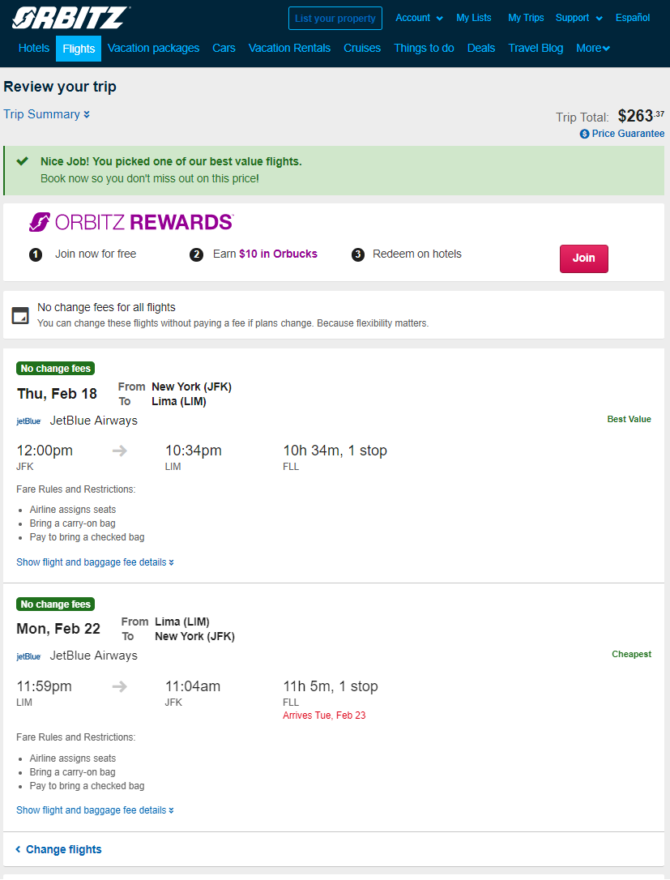In the detailed photographic image of a webpage, the interface is prominently branded at the top with a blue banner featuring the white text "Orbitz." The banner includes navigational options such as "List Your Property," "Account," "My Lists," "My Trips," and "Support," along with light blue subheadings labeled "Hotels," "Flights" (which is highlighted in light blue), "Vacation Packages," "Cars," "Vacation Rentals," "Cruises," "Things to Do," "Deals," "Travel Blog," and "More."

Beneath the blue banner, the white background of the page displays a black heading reading "Review Your Trip." Accompanying this section is a "Trip Summary" header, marked with blue arrows pointing downward. The summary reveals a trip total of $263.37 and includes a "Price Guarantee" highlighted in blue. An eye-catching green banner states, "Nice job, you picked one of the best value flights. Book now so you don't miss out on the price."

Further down, in purple text, the "Orbitz Rewards" section encourages users to "Join now for free" and earn $10 in "Orbucks," redeemable at hotels. This section features a notable pink "Join" button. Additionally, the page details flight information with a green button labeled "Leaving from JFK to Lima."